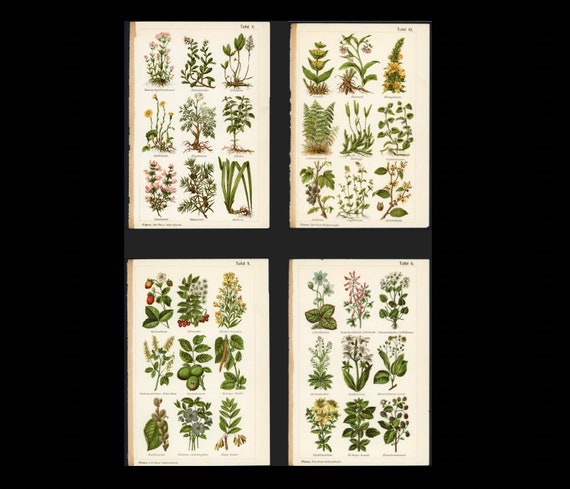This image showcases a striking collage of four botanical identification posters, elegantly displayed against a sleek black background. Each poster, created on canvas, meticulously illustrates nine distinct plants with vibrant, detailed, and colorful drawings. The background of the pages is a very light beige, and the edges of the canvases are visible, emphasizing their physical form. At the bottom of each plant drawing are their names, typed in very small black letters, making them hard to read from a distance. The plants, while diverse, predominantly feature green leaves, with many adorned with flowers in muted shades of yellow, pink, lilac, and blue. A few plants are purely leafy, including some that appear tree-like or fern-like. The overall presentation combines scientific precision with artistic charm, capturing the intricate beauty of each botanical specimen.